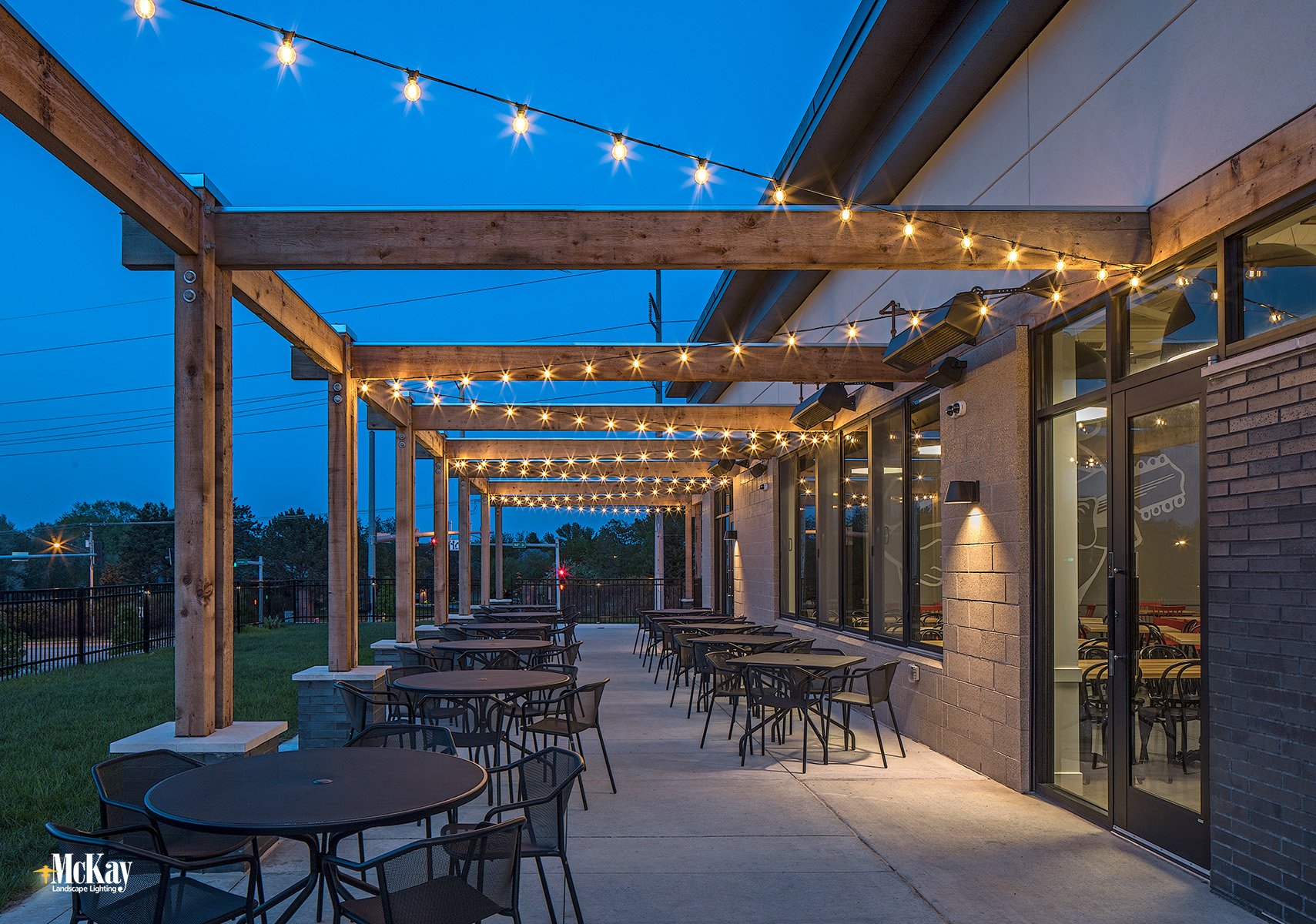The image depicts an outdoor patio area of a restaurant. This patio space, situated beside a brick-walled building, features uncovered wooden beams arranged in a saw-tooth zigzag pattern, adorned with string lights for illumination. These lights are likely to help guide diners, especially during the evening hours when the scene is captured—it’s around dusk, as indicated by the sky's deep blue hue and the low light conditions.

The patio is equipped with round, black, metal tables, each surrounded by four matching metal chairs. There are approximately 15 tables visible in the image. On the right side of the patio, a glass sliding door provides access to the indoor portion of the restaurant, where the decor transitions to rectangular, wooden tables.

While the patio offers a charming dining experience under the open sky, it lacks weather protection, such as fans or shade, which might make daytime dining uncomfortable on hot days. The bottom left of the image contains the text "McKay Landscape Landing," suggesting this is an advertisement for the company responsible for the patio's design, particularly its distinctive lighting setup.